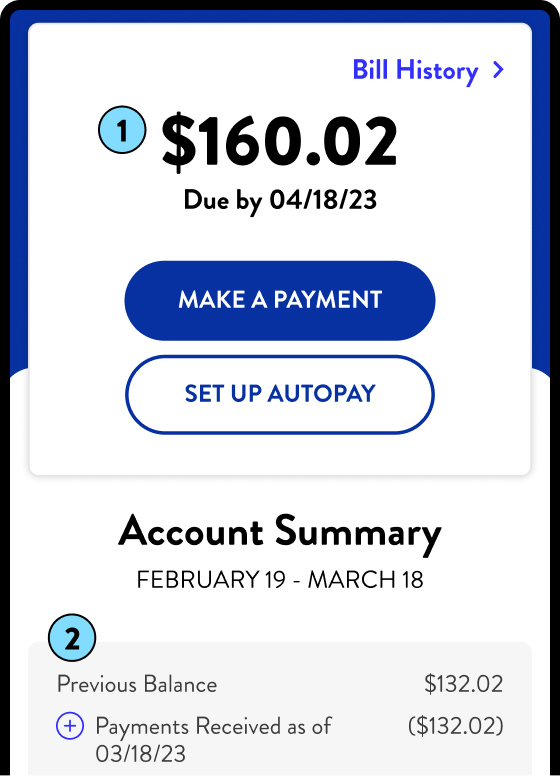The image depicts a screen from a payment service interface. The screen has a white background with a blue header at the top which indicates "Bill History" alongside a right-pointing arrow. Prominently displayed is a blue circle with the number "1" in black inside it, indicating perhaps the first item in a list.

Below this, it states an amount of "$160.02" due by "04/18/23". Two action buttons are present beneath this information: a blue "Make a Payment" button and a white "Set Up Auto Pay" button with a blue outline.

Further down, an "Account Summary" section highlights the billing period from "February 19 through March 18". Here, a blue circle with the number "2" provides additional details. The "Previous Balance" is listed as "$132.02". An adjacent circle with a plus sign indicates "Payments Received as of 03/18/23" totaling "($132.02)", showing the previous balance has been paid off. The current due amount of "$160.02" needs to be paid by April 18th.

Notably, the screen lacks any branding or specific indications of the payment service. The design prominently features a white background with elements in blue and black, organizing the billing information clearly and concisely for the user.